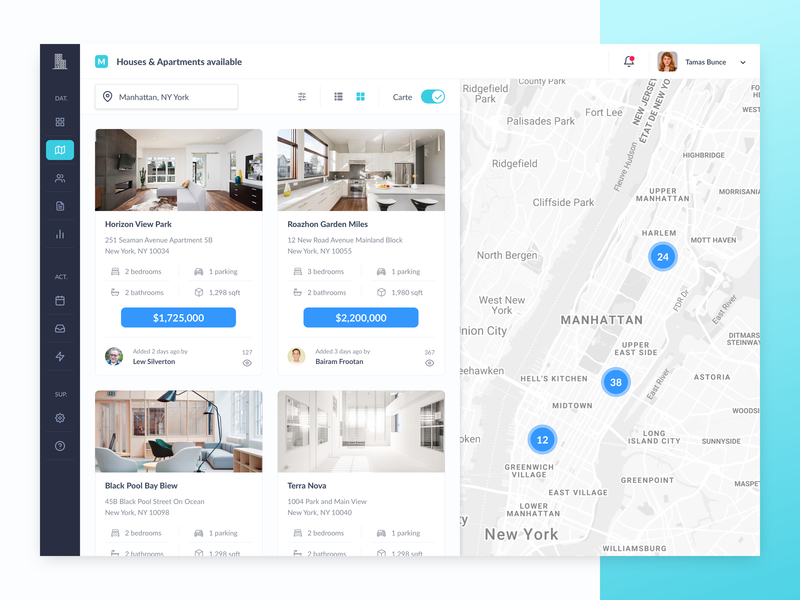A detailed list of residential properties in various neighborhoods of Manhattan, New York, is displayed in this image. It features a variety of apartments with specific details about each one:

1. **Aqua M on Seaman Avenue**:
   - Location: Apartment 5B
   - Layout: 2 bedrooms, 2 bathrooms
   - Amenities: One parking spot
   - Size: 1,298 square feet
   - Price: $1,725,000

2. **Raison Garden Mile**:
   - Location: New Road Avenue, Mainland Block
   - Layout: 3 bedrooms, 2 bathrooms
   - Amenities: One parking spot
   - Size: 1,980 square feet
   - Price: $2,200,000
   - Description: Very open with plenty of windows

3. **Blackpool Bay View**:
   - Location: Ocean (exact address unclear)
   - Layout: 2 bedrooms, 2 bathrooms
   - Amenities: One parking spot
   - Size: 1,298 square feet
   - Price: Not disclosed

4. **Terra Nova**:
   - Location: Park and Main View
   - Layout: 2 bedrooms, 2 bathrooms
   - Amenities: One parking spot
   - Size: 1,298 square feet
   - Price: Not disclosed

Additionally, the image shows a map of New York with specific markers:
- A blue circle marked '24' near Harlem
- A marker '38' by Hell's Kitchen
- A marker '12' by Greenwich Village

The correlation of these markers to the properties listed is not made clear in the description.